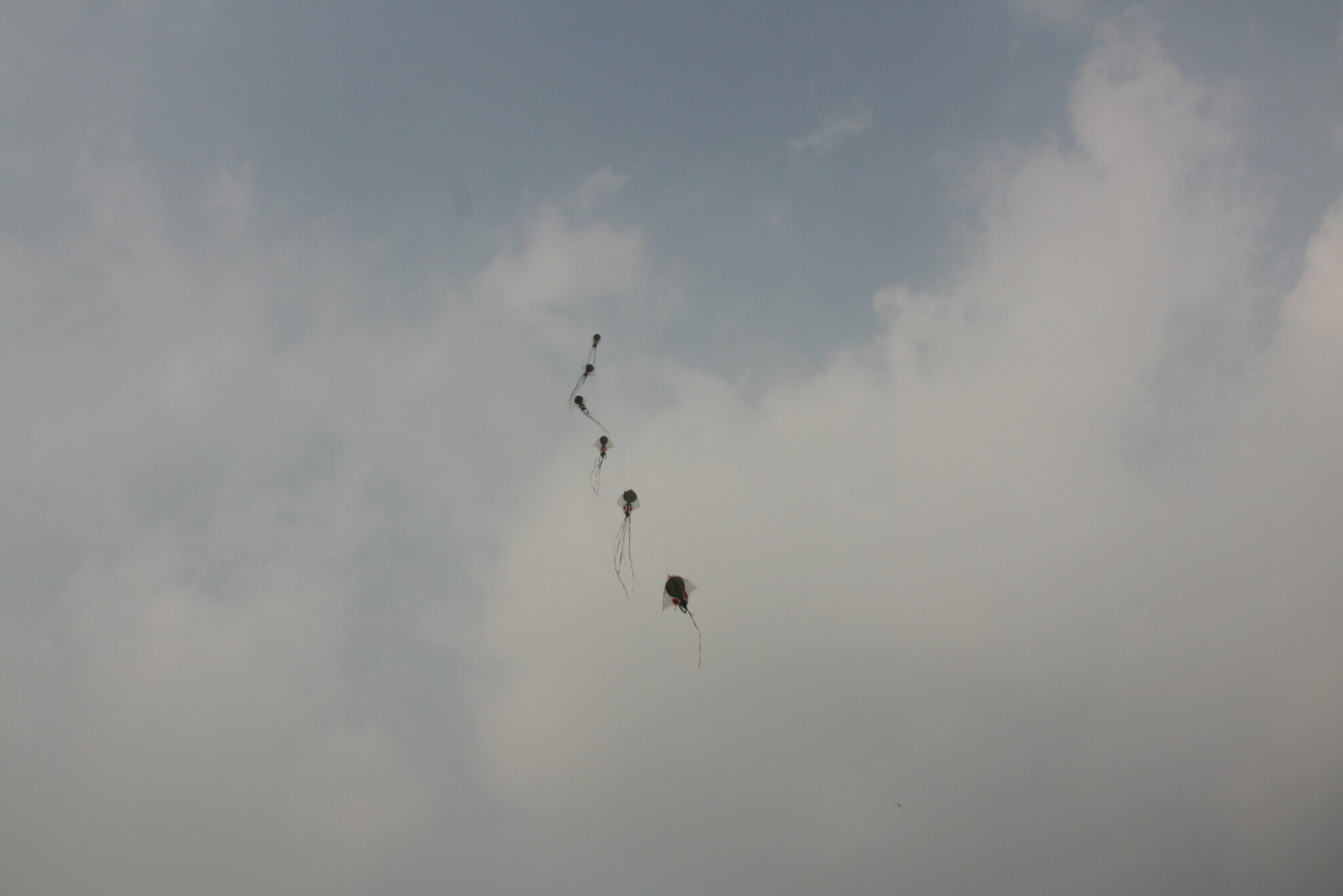In this image, the sky is predominantly covered with grayish-white clouds, filling the bottom two-thirds of the scene, creating a muted, overcast ambiance. Dominating the center of the picture are six enigmatic objects, arranged in a straight line ascending towards the sky. These objects are difficult to identify precisely, with various similarities to kites, insects, or perhaps other flying creatures. Each one exhibits a distinctive shape, featuring a large, almost peanut-shaped body that narrows in the middle and expands at the sides, paired with long, trailing limbs or strings. The shapes are reminiscent of jellyfish, with their triangular wings or kite-like forms and stringy appendages. The alignment magnifies their perspective, as the topmost object appears much smaller, enhancing the sense of depth and height within the cloudy expanse.